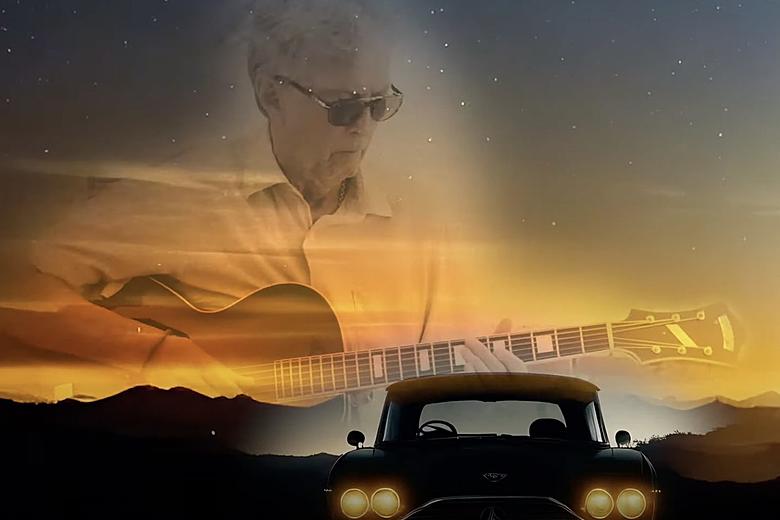In a digitally rendered, horizontally oriented image, an older gentleman with white hair and clad in a short-sleeved, white button-up collared shirt and dark sunglasses plays an acoustic guitar. His transparent, superimposed image hovers against a dark, starry night sky that transitions into a pale yellow sunset near the silhouetted mountain ranges below. The man’s concentrated gaze is fixed on his fingers as they strum the black guitar. In the foreground, an old-timey black sedan, possibly from the 1940s or 1950s, stands facing away towards the distant landscape, its taillights and two pairs of headlights—now warm-colored—casting a glow on the dark roadway. The composition evokes a sense of reflective nostalgia, as if depicting the sunset of the musician’s career.